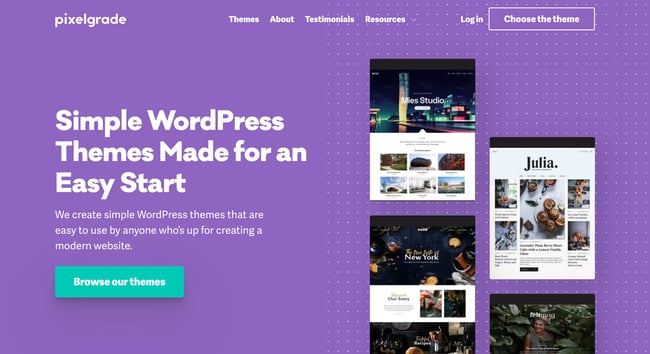This landscape image appears to be an advertisement for a company named Pixel Grade, prominently featured in white text at the top left. The background has a deep purple hue, with the left half being solid and the right half adorned with small, faint white dots arranged in a vertical polka dot pattern. The left side of the ad emphasizes the company's tagline, "Simple WordPress themes made for an easy start," with a green button below it that says "Browse our themes." 

On the right side, various example themes are showcased in images. The topmost theme, labeled "Me Studio," features a cityscape. Below it, another theme titled "Julia" displays food imagery. Further down, a theme named "New York" also seems to focus on food, although the details are somewhat unclear. The bottom theme shows a woman amidst leaves. Above these themes is a navigation bar listing subcategories: themes, about, testimonials, resources, login, and a button labeled "Choose the theme."